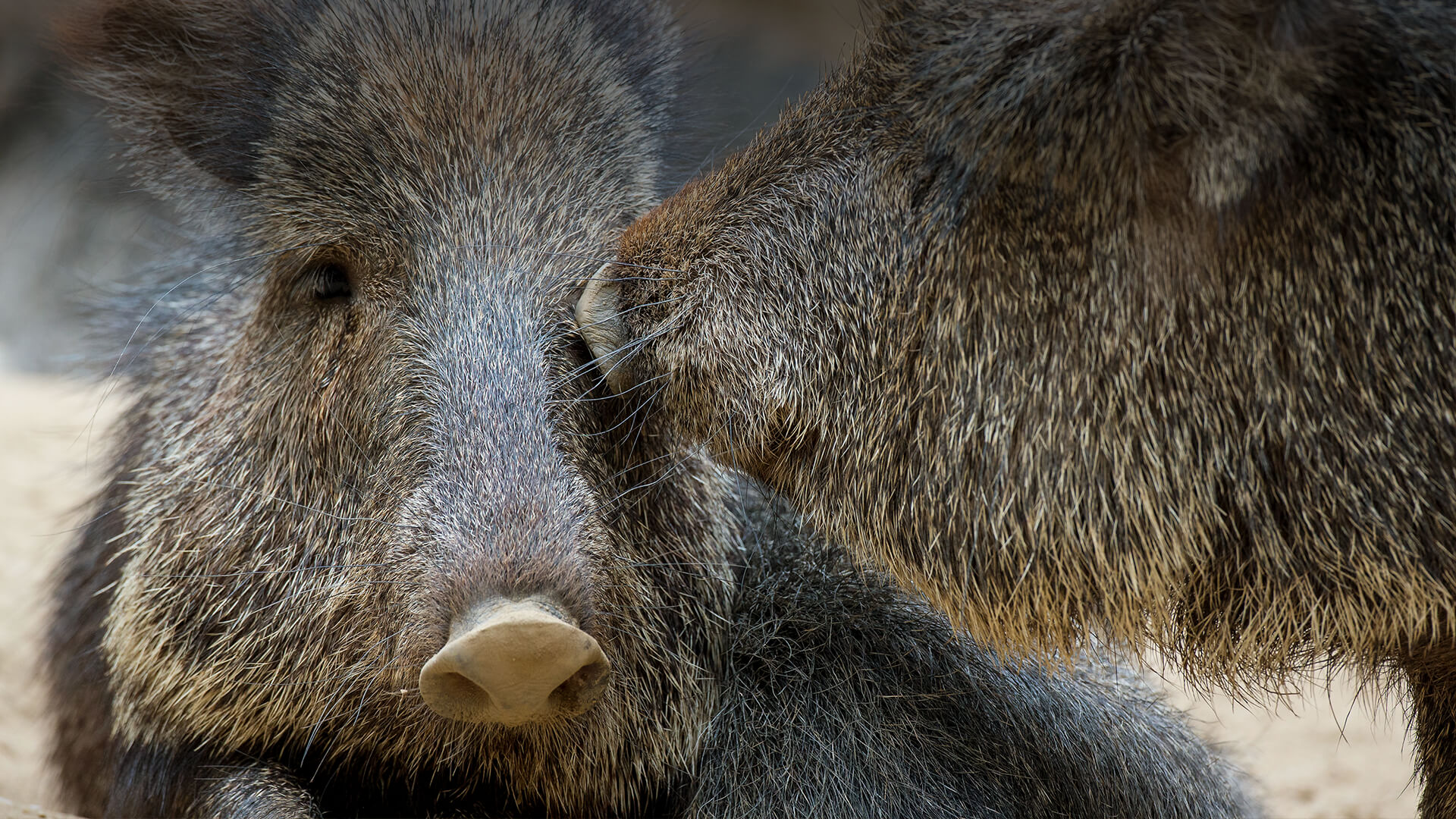The photograph captures an intimate, close-up scene of two boars. The boar on the right side of the frame has a prickly, brown coat with light brown and gray accents, and it is oriented with its head facing left. Its beige, flat snout is touching the area near the eye of the other boar. The second boar, positioned on the left and facing forward, has a fuzzy, brown head and a light brown snout. A small dark spot that resembles an eye indicates it might be resting. Although the background is mostly blurry, there is a light brown surface beneath them, and the scene evokes a sense of closeness and affection between the two animals. The photograph highlights their coarse, grayish-brown fur and distinctive features, lending a sense of warmth and connection in their interaction.